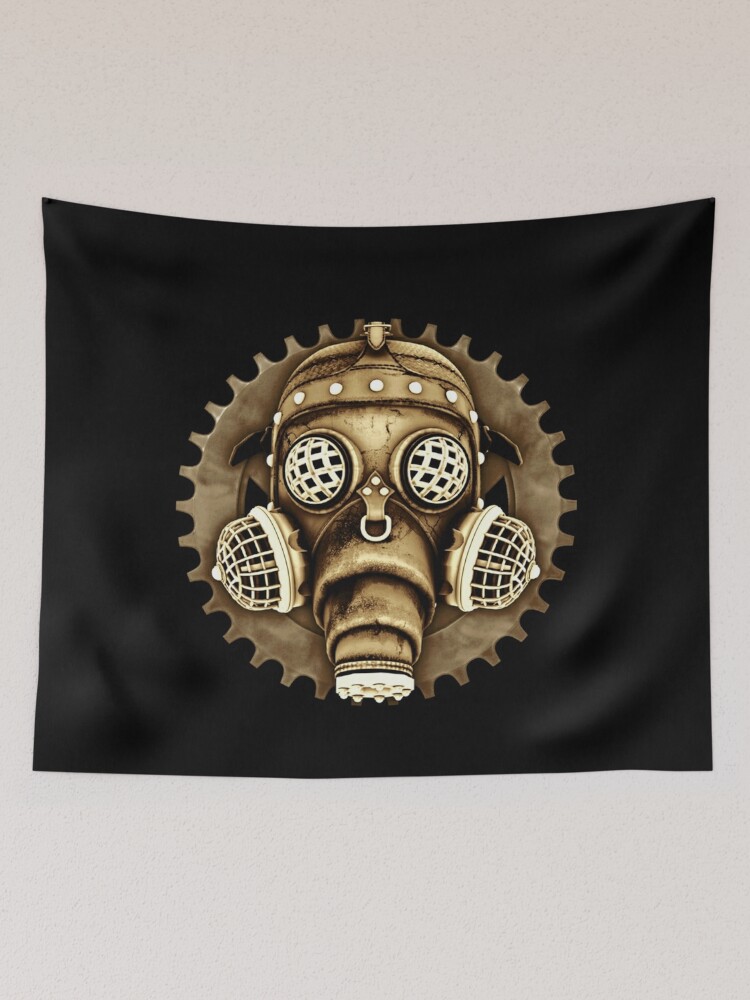In this photograph, a black flag hangs against a white or off-white wall. The flag, nearly square-shaped, features a prominently centered design that resembles an industrial-era gas mask, crafted from bronze-colored parts. The gas mask has a number of intricate details, including a flexible, collapsible ventilator hose attached to its mouth, ending in a cylindrical canister. The cheeks of the mask each have raised respirator shapes with mesh-like coverings, which are repeated over the eye holes. Surrounding the gas mask, there's a large circular gear or saw-blade-like design in a dark gray or copper color, adding an industrial flair. The mask's eyes have a light beige, checkered appearance resembling flypaper, and the design is further detailed with studs around the top of the mask. This flag is both strange and elaborate, combining elements of vintage machinery and gas masks into a striking visual.